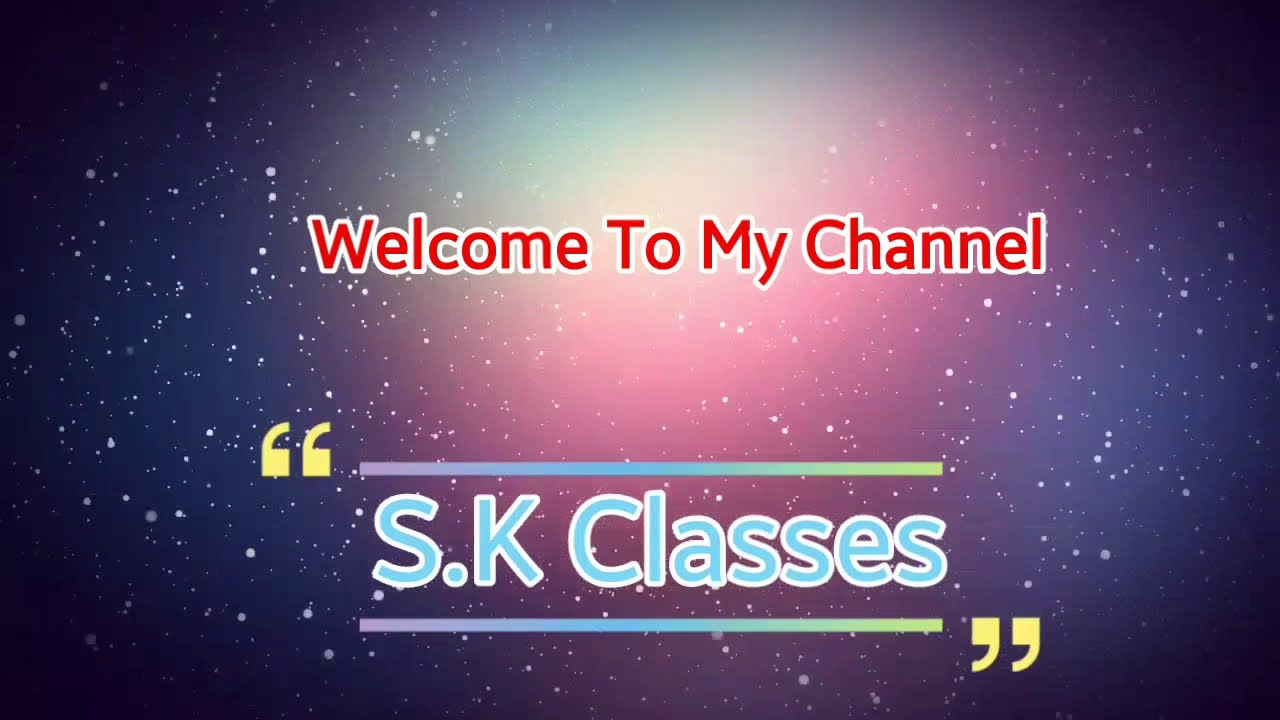The rectangular image features a cosmic outer space background with a starry field that progresses from dark black at the edges to a vibrant, glowing center. This central area is a bright cloud of pink, blue, and light green hues, giving it a rainbow-like appearance. Overlaid on this backdrop, the top-centered text "Welcome to My Channel" is prominently displayed in red Times New Roman font, bordered by a white outline. Below this, there are yellow quotation marks on either side of the phrase "S.K. Classes," which is written in turquoise and similarly outlined in white. This text is flanked by two horizontal lines above and below, which transition in color from purple on the left, to blue in the middle, and finally to green and yellow on the right.